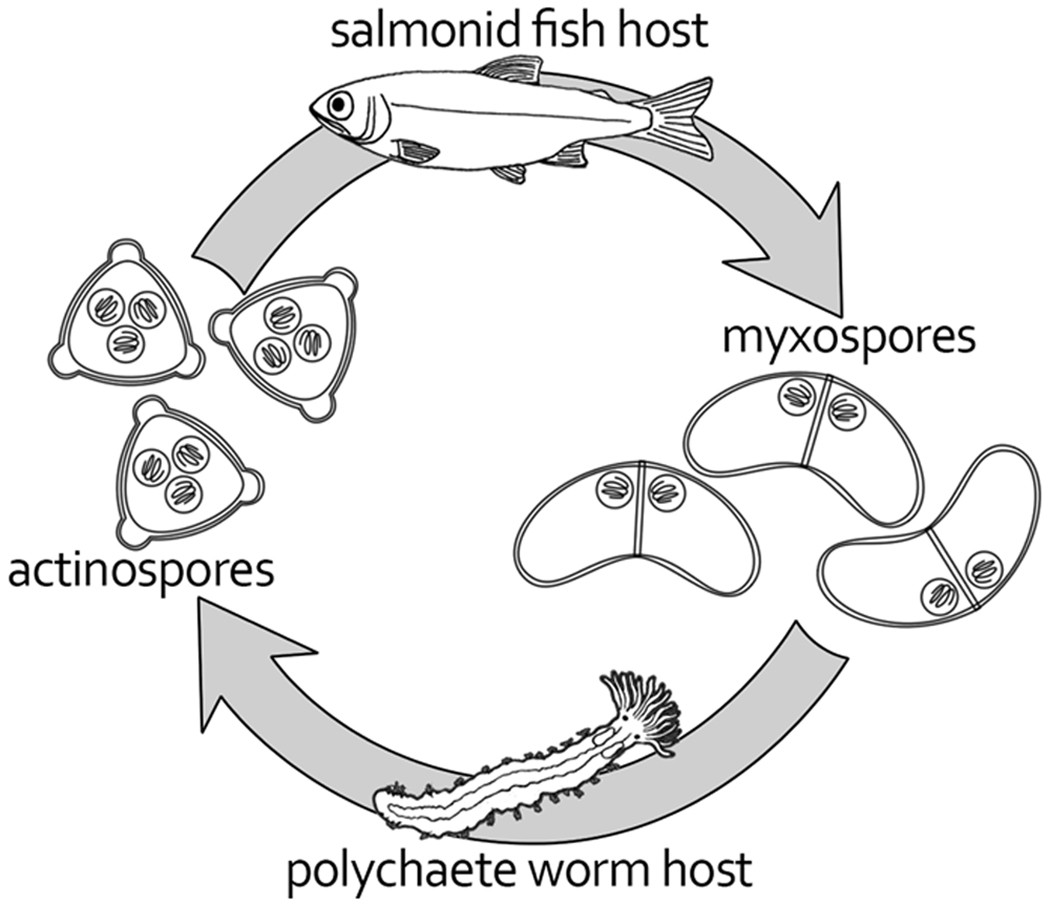This black and white scientific diagram, likely sourced from a biology textbook, illustrates the life cycle of parasites involving a Salmonid fish host and a Polychaete worm host. The diagram is arranged in a circular, clockwise motion, denoted by curved arrows. At the top, a fish is labeled "Salmonid Fish Host," initiating the cycle. To the right, kidney-shaped structures labeled "Myxospores" feature vertical lines and paired internal circles. Below, a long, narrow worm with a brush-like end is labeled "Polychaete Worm Host." Finally, towards the left, three rounded triangular shapes labeled "Actinospores" contain dots with internal scribbles, completing the cycle before returning to the Salmonid fish host. The diagram uses shades of gray and white line sketches to represent the various stages and hosts involved.